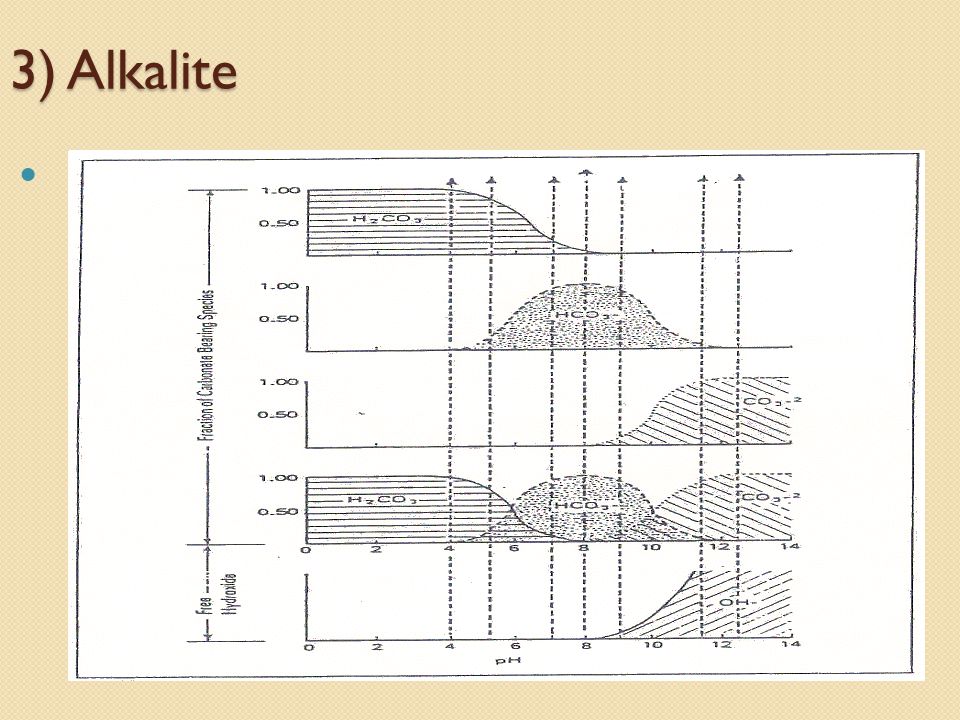The image features a light brown background with the number "3" in the top left corner, followed by a parenthesis and the word "Alkalite" in a brown or maroon font. Directly beneath "Alkalite" is a small blue dot. The main focus of the image is a white rectangular piece of paper that appears to have been scanned. The paper contains a series of black and white graphs and charts with lines that slope upwards and downwards, indicative of some kind of measured data. Arrows pointing upward and labels such as "fraction of carbonate bearing species" and "free hydroxide" are visible, alongside numerical notations. At the bottom of the charts, "pH" is indicated, adding context to the nature of the data being presented.